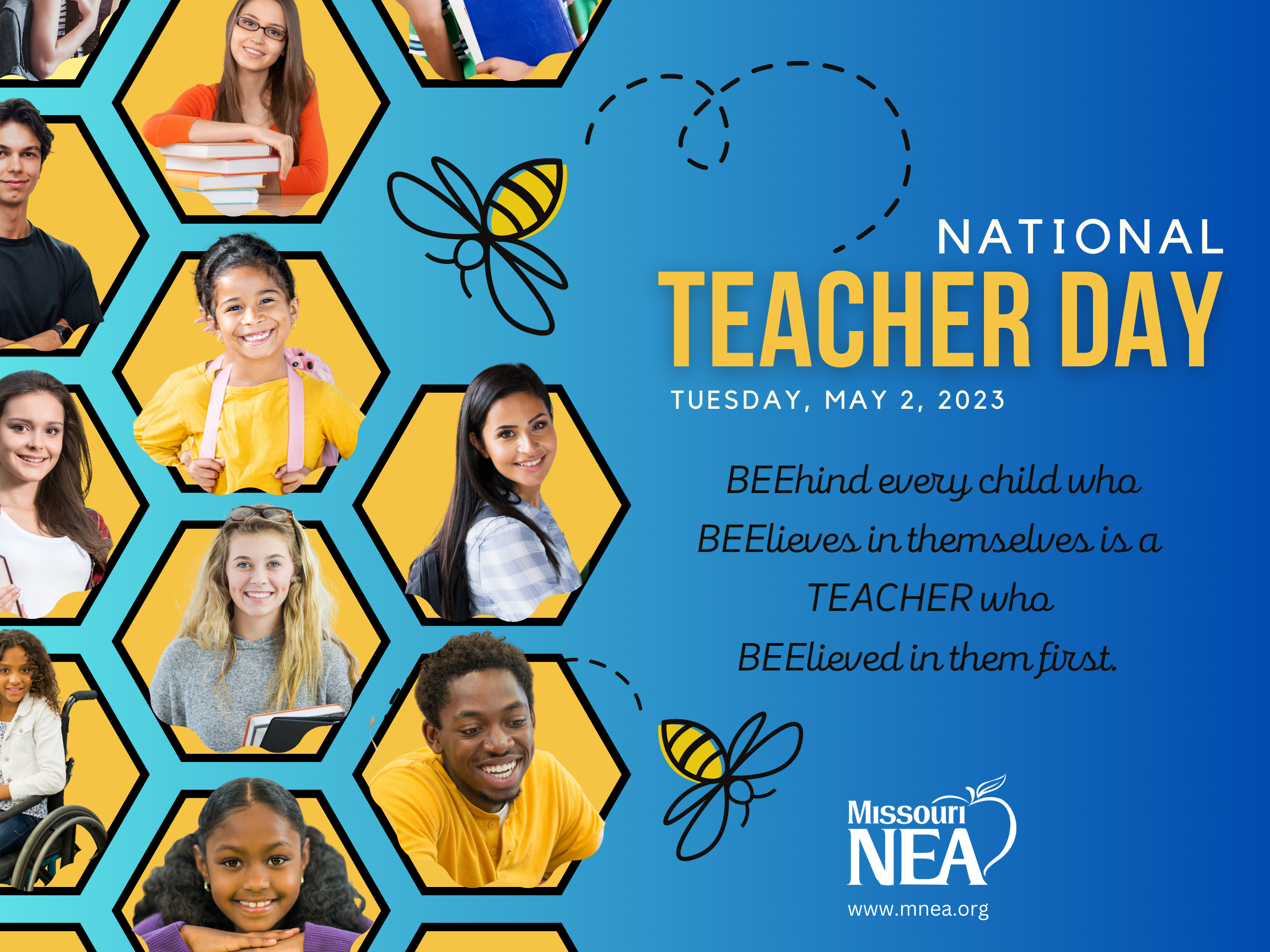The image is a detailed poster for National Teacher Day, held on Tuesday, May 2, 2023. The background is blue, creating a calm and inviting atmosphere. The left side of the poster features several young students and teenagers within yellow hexagonal boxes, reminiscent of a beehive. Adding to this bee theme, small illustrated bees are flying around the hexagons. On the right side, the main heading, "National Teacher Day," is displayed prominently in large gold-yellow text. Below this, a poignant message reads: "Behind every child who believes in themselves is a teacher who believed in them first." The words "believes" and "believed" are creatively spelled with an extra 'E', forming 'BEE-lieves' and 'BEE-lieved,' accompanied by bee illustrations. At the bottom of the poster, the logo for Missouri NEA is visible, along with their website, www.mnea.org, in white text.